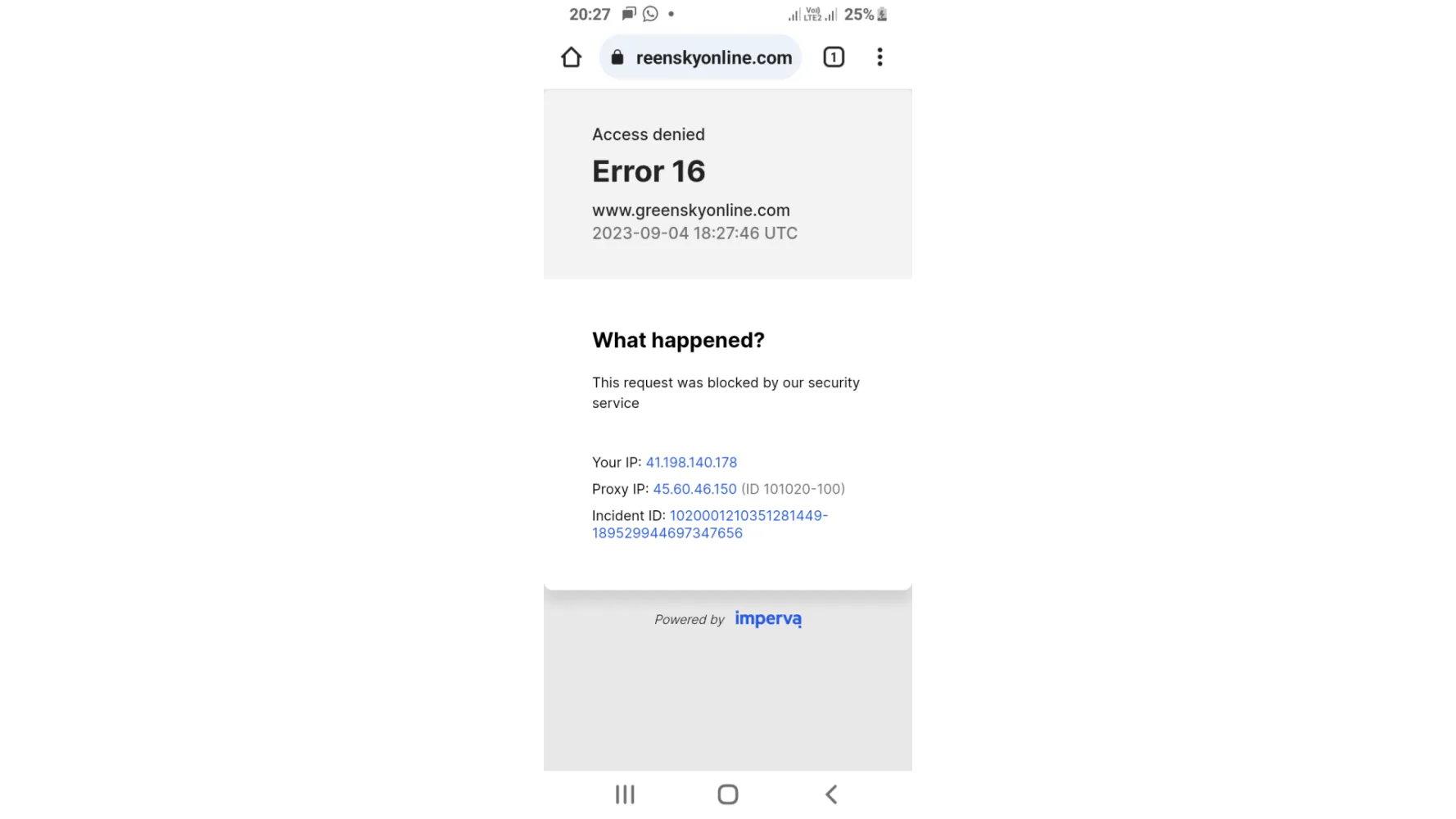This image is a compact screenshot captured from a mobile device, showcasing a webpage with an error message. At the top, within a white banner, the address bar is visible, featuring a lock icon followed by the URL "R-E-E-N-S-K-Y online.com" in black text. To its right, a square icon displays the number one, while a home icon is positioned to the left. In the upper left-hand corner, the time is shown as 20:27. The battery indicator in the upper right-hand corner reveals that the device's battery is at 25%.

The primary content of the screenshot is organized into three sections with a gray-white-gray color scheme. The first gray section features the message "Access Denied, Error 16," along with the URL and a timestamp "2023-09-04, 18:27:46 UTC." The middle white section contains the text "What happened?" followed by an explanation stating, "This request was blocked by our security service." This part also lists the user's IP, proxy IP, and incident ID, with each field followed by a series of numbers highlighted in blue font.

At the bottom, another gray section includes the phrase "Powered by Imperva," where "Powered by" is italicized in gray, and "Imperva" is prominently displayed in blue. Finally, the screenshot concludes with the standard three bottom navigation icons found on mobile devices, situated at the very bottom of the screen.